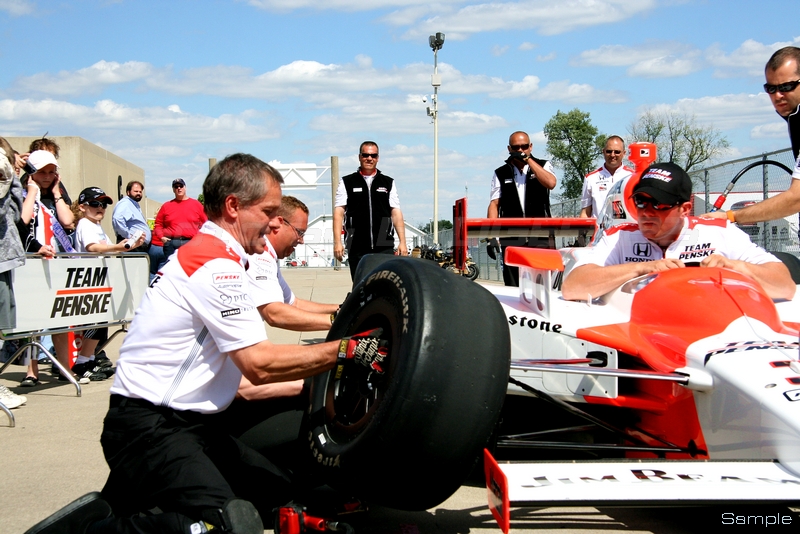This photograph captures a bustling pit stop at a professional car race event featuring a sleek, white and red, aerodynamic racing car with a prominent rear spoiler and massive black tires devoid of tread. In the center of the image, mechanics clad in white collared shirts and black pants, adorned with various sponsor logos including Firestone, Honda, and Team Penske, diligently work to replace or fix a tire. The driver, distinguishable by his black cap and sunglasses, is slightly to the right of the image, closely observing the procedure, possibly holding the tire or preparing to install a new one. The scene is set on a sunny, clear day with blue skies and a few white clouds visible, casting a bright yet calm atmosphere over the event. In the background, spectators, including children, stand behind a barrier marked "Team Penske," eagerly watching the action unfold. To the left, a building and some trees are visible, adding context to the location, while a chain-link fence and light gray asphalt define the racing environment on the right.